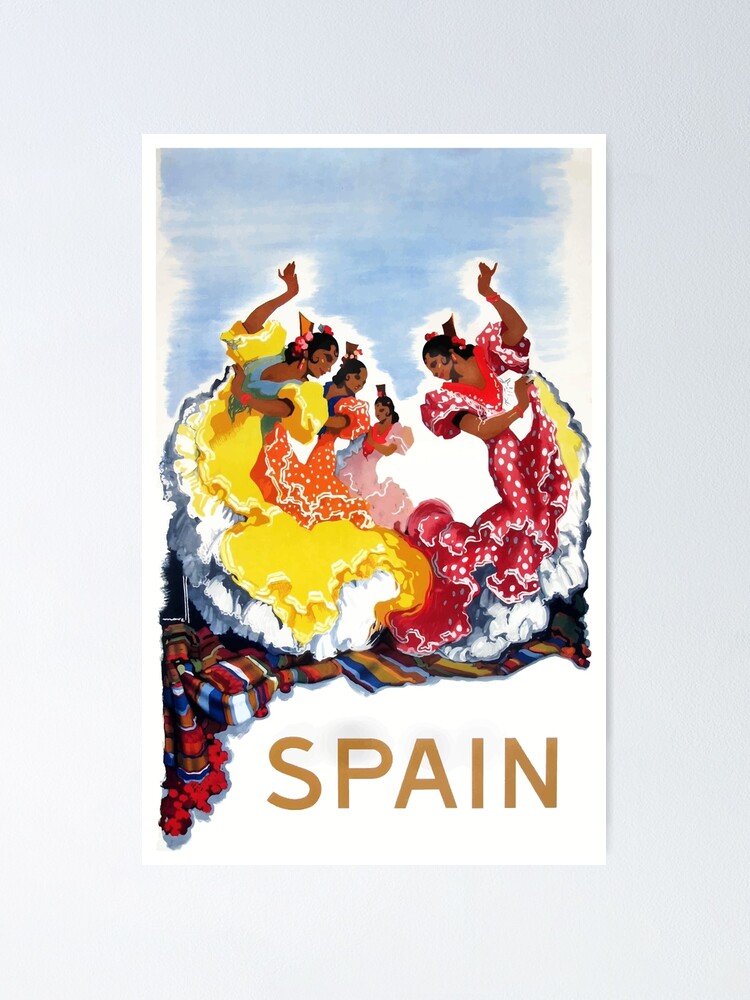This is a detailed travel poster for Spain featuring an animated painting of festive, dancing women against a beige background. The artwork is framed with a gray matting and a small white border, and it features the word "SPAIN" in bold, brown capital letters at the bottom right. 

The scene depicts four women engaged in what appears to be a traditional flamenco dance. They are adorned in colorful, ruffled gowns: one in a frilly, elaborate Spanish-style dress with flowers in her slicked-back black hair, another in a peachy polka-dotted dress, a third in a pink dress with a similar hairstyle, and the last in a pink dress with red polka dots, holding up her skirt to reveal a yellow-frilled underskirt. Some of the women have their arms raised gracefully in the air amidst a backdrop that suggests a serene blue sky. The composition and vibrant attire reflect the lively and culturally rich essence of Spain.